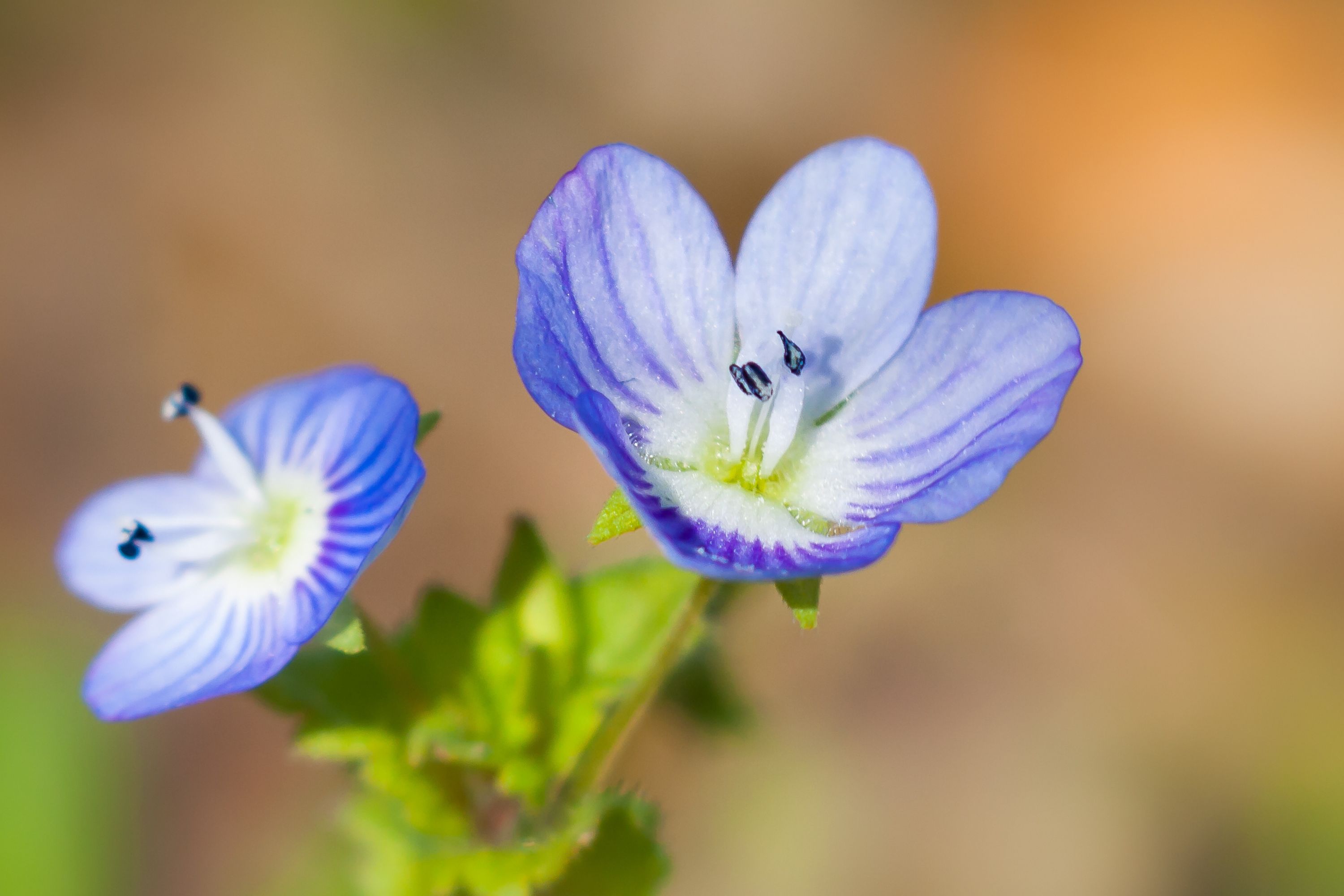This image captures an intricate close-up of two connected flowers on the same green stem, set against a blurred, muted background of beige, gold, brown, and green hues. Each flower features a visually striking gradient, with a white center transitioning to a bluish-purple that deepens at the petal edges. The central area of each flower is marked by fine green pistils with tiny black tips. Surrounding these blooms are bright green leaves, adding further detail to the composition. The photograph's sharp focus on the flowers accentuates their delicate, natural beauty while rendering the surroundings softly out of focus, highlighting the vivid and realistic details of these wilderness blossoms.